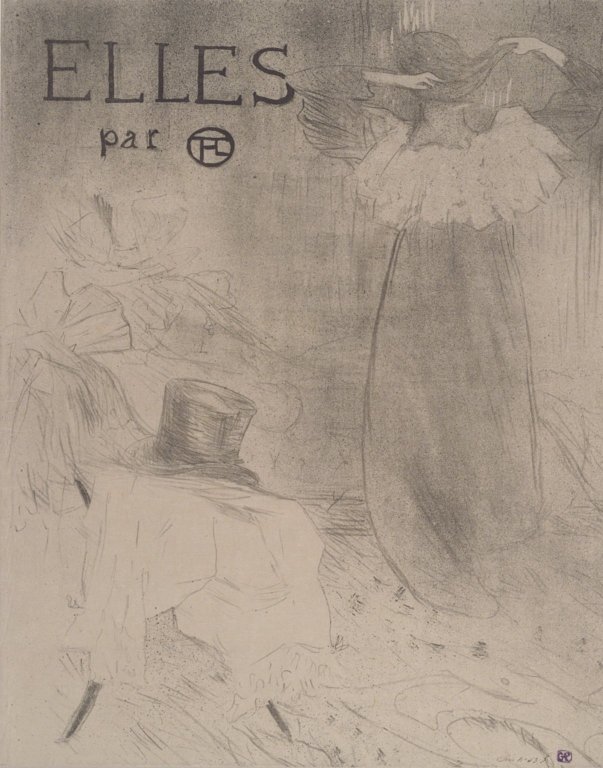This image showcases an intricately detailed pencil sketch dominated by shades of black, gray, and light white. On the right side, there is a striking figure of a woman seen from behind. She wears a floor-length, dark-colored nightgown or dress with a frilly neckline and a white collar. Her long sleeves cover her arms, which are bent at the elbows as both hands run through her hair. 

To the left of the woman, a top hat rests atop what appears to be a piece of folded fabric or possibly a shirt draped over a chair. Above this, in the top left corner, the text "Elles" followed by "par" sits alongside a circled logo composed of lines. This area carries an air of elegance and mystery, adding depth to the overall composition. Despite the difficulty in discerning finer details, such as the tiny, indistinct signature in the bottom right, the sketch beautifully balances various elements and textures. Overall, the scene feels like an artist’s sophisticated tribute, potentially worthy of a comic book cover or a fashion illustration, showcasing a blend of intricate design and captivating narrative.